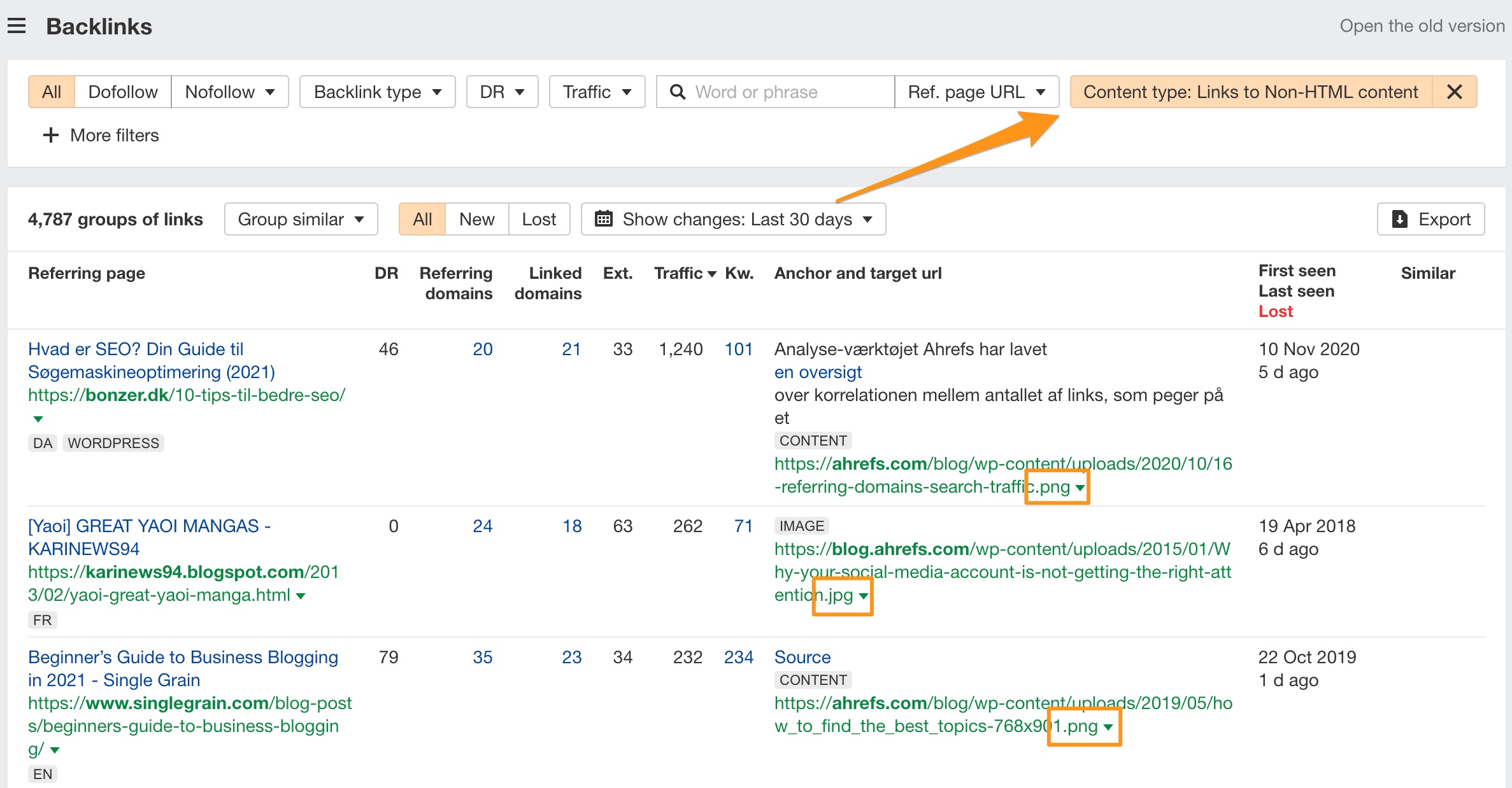The screenshot depicts a detailed section of a website related to backlinks analysis. At the top, there's a banner featuring a hamburger menu icon on the left—a set of three horizontal, evenly spaced lines. Adjacent to this icon is the word "Backlinks" in a larger font with a capital 'B.' To the right of this, a clickable text reads, "Open the old version."

Below this top banner, there is a white menu bar that spans horizontally and includes filter options labeled "All," "Do Follow," and "No Follow," all in black text. The "All" option is highlighted with a peach background. Further to the right, there is an additional filter button labeled "Plus More Filters."

Beneath this bar is a series of dropdown menus titled "Backlink Type," "DR" (Domain Rating), "Traffic," and "Ref.PageURL," each allowing for more specific filtering. There’s also a search bar with a magnifying glass icon labeled "Word or Phrase," alongside another dropdown for "Peach Contact Type" and another filter labeled "Links to non-HTML content" which has an 'X' indication to clear the filter.

An orange arrow points towards the peach-colored space with text inside it. Below this section is a white background area displaying the text "4,787 groups of links," along with additional filtering options for grouping similar links, selecting all, new, or last. A calendar icon with a dropdown menu allows the viewer to show changes over the last 30 days. 

At the very bottom, more descriptive filters include options for "Referring Type," "DR," "Referring Domains," "Linked Domains," "EXT," "Traffic," "KW," "Anchor," and "Target URL."